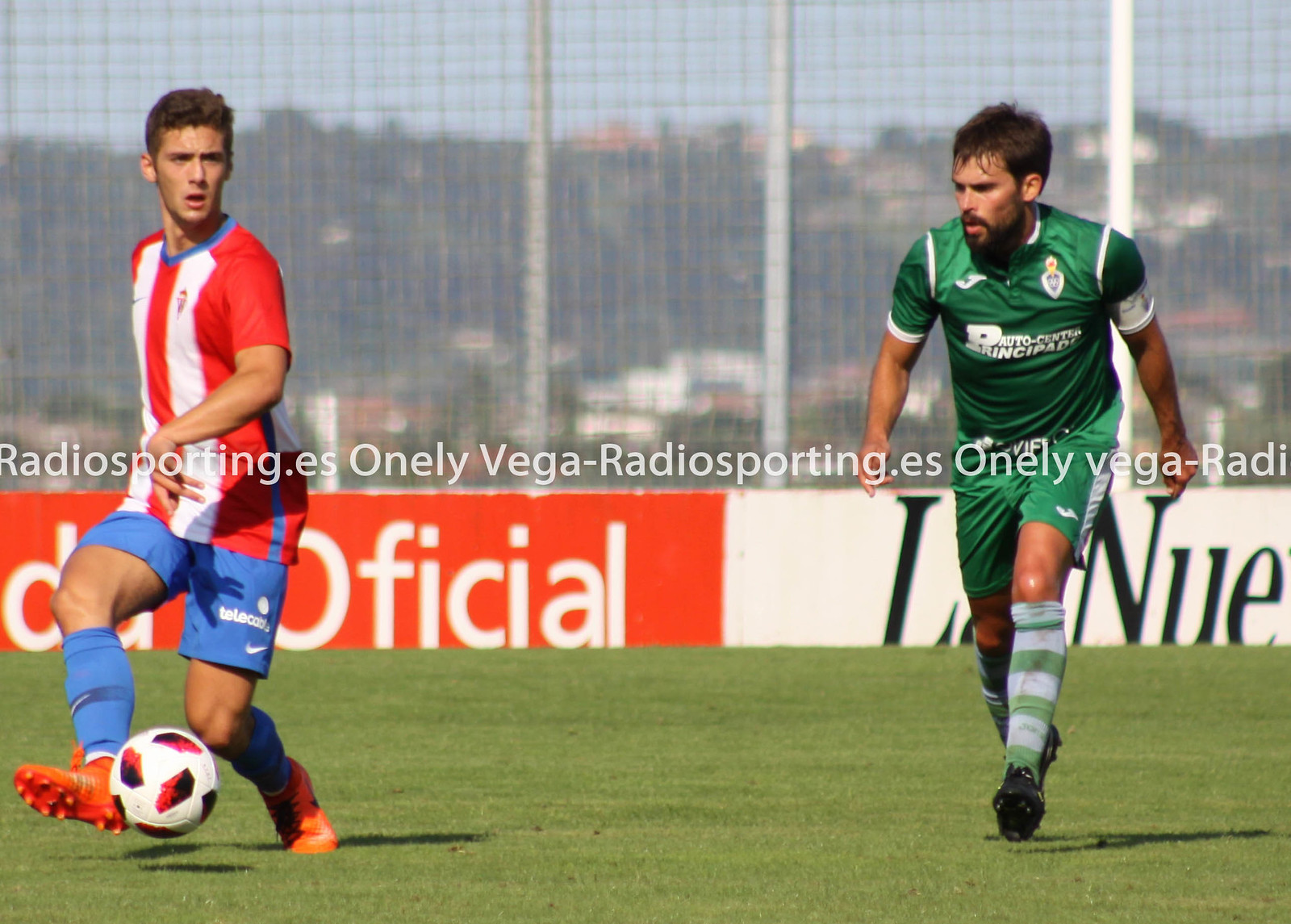In this dynamic image set on a green grassy soccer field, two men are captured in the heat of action. The man on the left is in the midst of kicking a white soccer ball adorned with red and black panels. He dons a vertically striped red and white jersey with a light blue collar, paired with blue shorts and tall blue socks. His bright orange soccer shoes stand out, and his short brown hair and light skin are clearly visible. Chasing after him is another man clad in a green jersey with matching shorts. His socks, bearing light blue and green stripes, extend high up his legs, and he sports black soccer shoes. He also has short brown hair that appears wet and tanned skin. The backdrop features a large mesh netting fence with a red advertisement reading "Officiel" and other unreadable signs.